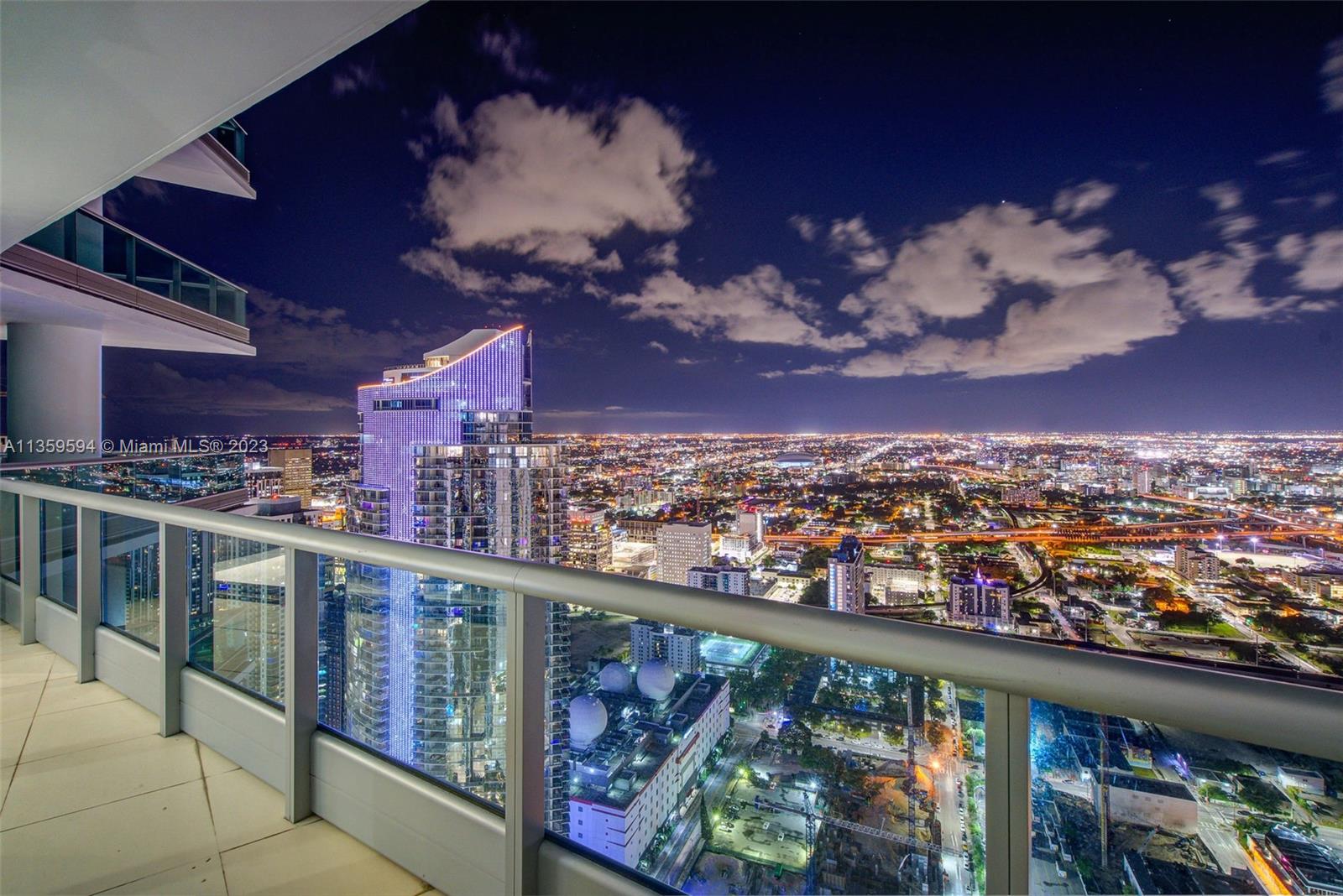This photograph captures a vibrant, bustling cityscape at night, dominated by the glittering lights and towering buildings that evoke the atmosphere of Miami, as confirmed by small text on the left indicating "Miami MLS 2023." The scene is viewed from a high-rise balcony, at least 40 stories up, giving a sense of both the immensity and the energy below. The silver railing of the balcony, designed with glass panels for an unobstructed view, frames the foreground where tan-colored tiles provide a quiet contrast to the city's liveliness. To the left of the image, part of another large building looms into view, hinting at vertical density. Above this, additional floors and balconies extend upwards, cementing the scene’s high-altitude perspective. The sky, a dark navy blue speckled with clouds, suggests early evening, adding to the dynamic yet serene ambiance of the photograph. Despite the city's urgency and busyness below, the balcony offers a peaceful, elevated vantage point, creating a unique juxtaposition that feels both urgent and tranquil.